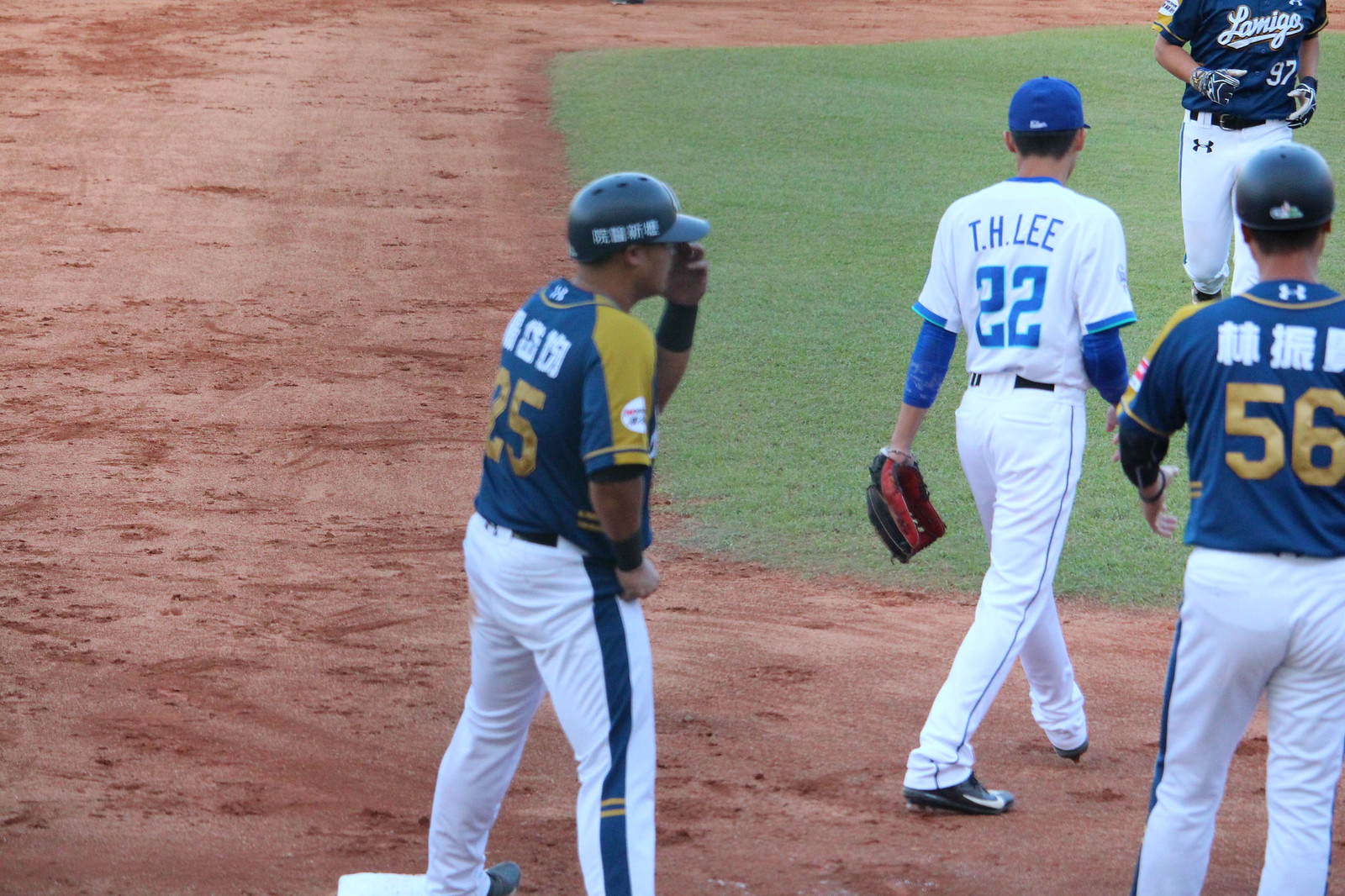The image captures a segment of a baseball field featuring four players, each wearing uniforms and gear that offer specific details. In the foreground stands a player on a base, dressed in long white pants and a distinctive blue and gold t-shirt with the number 25 on it. He wears a mostly gray baseball helmet adorned with white Asian letters. To his right is another player in white pants and a white jersey marked with "T.H. Lee" and number 22. This player sports a blue cap, a blue long-sleeved shirt underneath, and a glove on his left hand. Further to the right is a third player, also in white pants, wearing a dark blue shirt with the number 56. In the background, moving towards the group, is a fourth player, visible from the shoulders down, dressed in similar white pants and a dark blue t-shirt that prominently displays "LAMIGO" and the number 97. The carefully manicured field features clay dirt and grass, suggesting an engaging moment in what appears to be a baseball game between two Asian teams, inferred from the Asian writing on the jerseys.